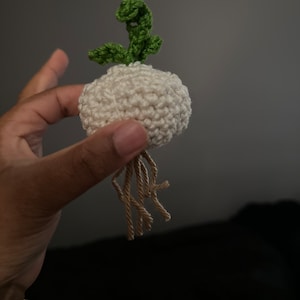The image features a left hand with a tanned skin tone, holding a handcrafted object illuminated against a dimly lit background. The hand, with a lighter underskin, showcases a small blemish on the first knuckle crease of the index finger. The object, gripped between the thumb and forefinger with the middle finger visible behind, appears to be a crocheted or knitted radish or turnip. The crafted vegetable has a bulbous, circular shape made of white yarn, with three green knitted leaves sprouting from the top and several grey yarn strands resembling roots hanging from the bottom. The background consists of a grey wall and a dark-colored piece of furniture, adding to the dim atmosphere of the photograph.